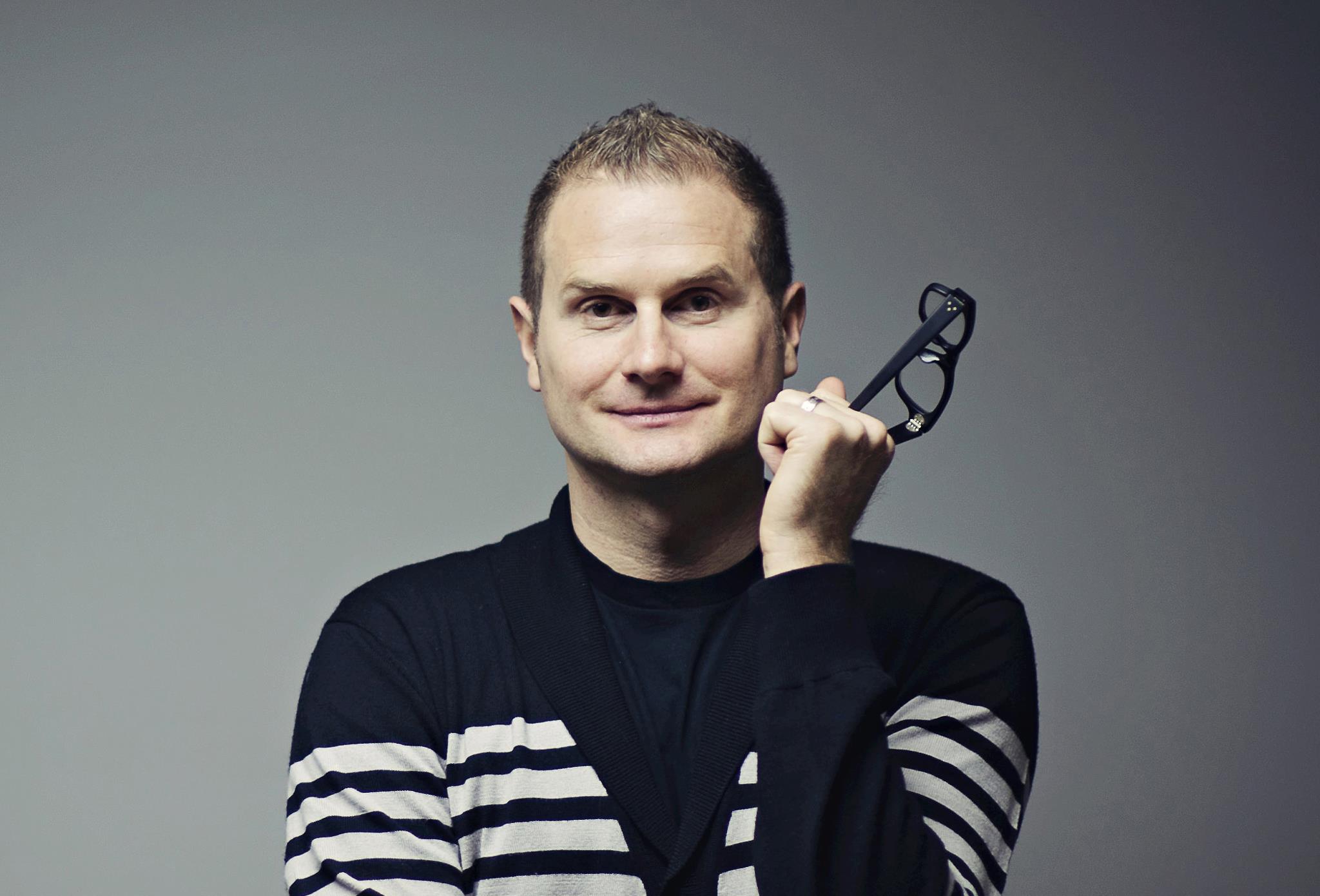A man is depicted in the image, dressed in a sophisticated combination of a black sweater layered over a black shirt. The sweater, which may also be referred to as a shawl, features an interesting design a little further down where it transitions into a white pinstripe pattern with black stripes interspersed. The man is holding a pair of black-framed glasses with square, almost oval-shaped lenses. His hairstyle is notably short, with a slight spike in the center and neatly combed sides. His facial expression exudes a sense of happy contentment, with a subtle smirk accentuated by slightly raised eyebrows and a few delicate forehead wrinkles. He has expressive brown eyes and a meticulously groomed, closely shaved mustache and beard.